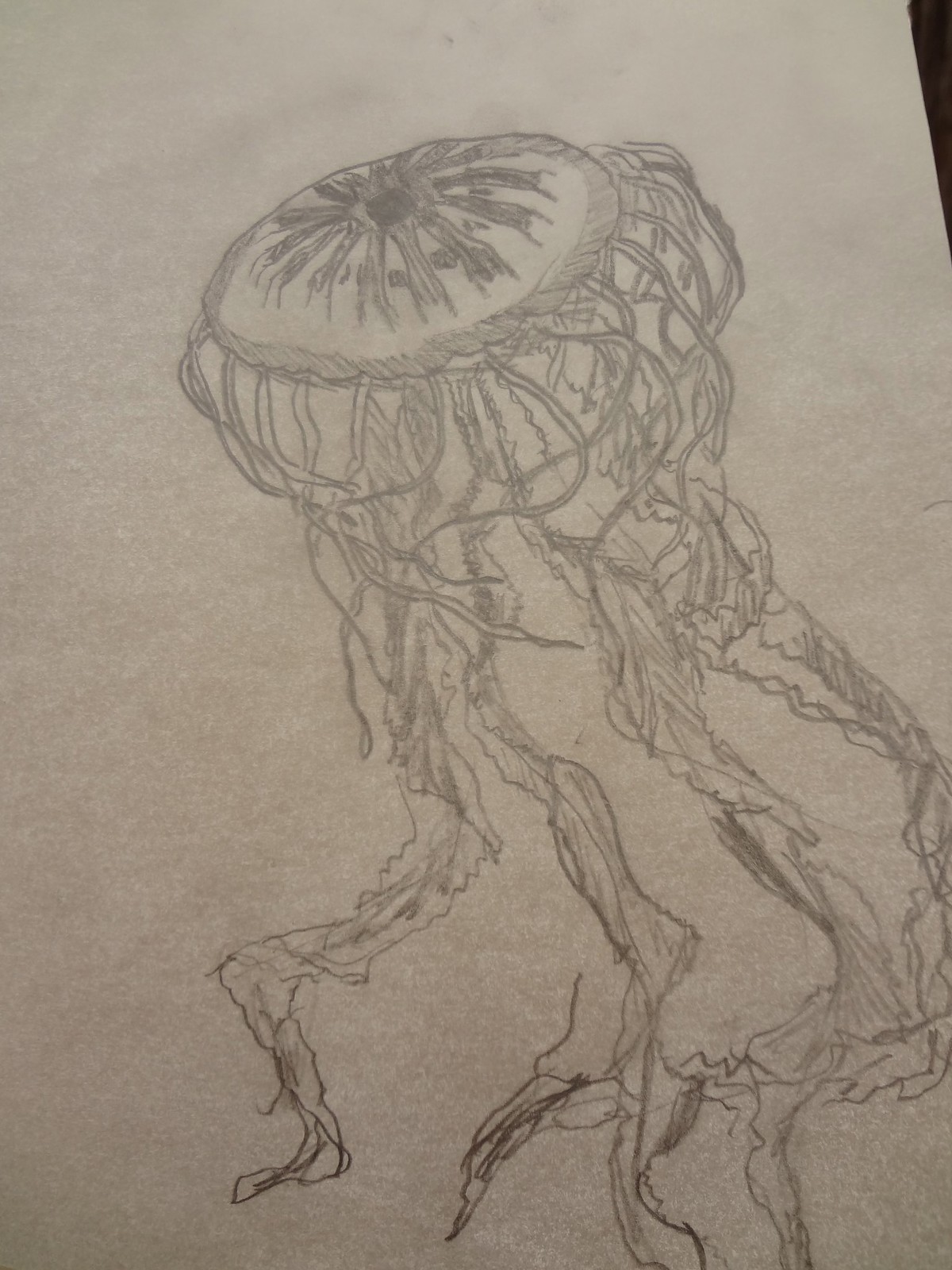This is a detailed, pencil-drawn image of a jellyfish on thin, off-white or grayish art paper, possibly tracing paper. The central feature at the top of the drawing is a relatively flat, circular body that seems to include an inner circle, perhaps representing the jellyfish's nucleus or brain, emphasized with shading around its inside edge. From this central circle, long, wavy tentacles flow downwards, comprising approximately 30 individual strands. These tentacles vary in length and have a distinct sinuous quality, often curving left and right, with some ending in foot-like shapes. The tentacles are depicted with detailed line work, enhancing the depth and texture, faithfully capturing the delicate stingers of the jellyfish. The image is notably detailed for a pencil drawing, with no accompanying text.